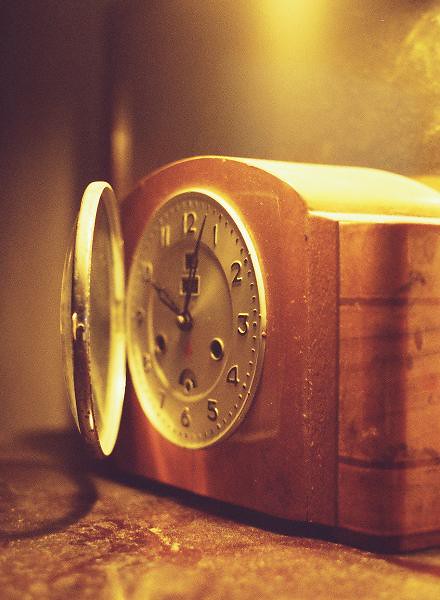This color photograph features a close-up of a small, vintage wooden clock designed to rest on a desk. The clock's face, adorned with gold elements, is meticulously captured with its glass covering opened, revealing the intricate details inside. The hour hand is pointing at 10 while the minute hand rests slightly after 12, indicating the time as 10:04. Above, a warm yellow light casts a golden glow, enhancing the clock's antique appeal and adding an artistic, almost nostalgic atmosphere to the scene. The clock's wooden frame is prominent, stretching from the center right to the left of the image. Additional details include a square section behind the minute hand for a key and three small winding circles at the bottom of the clock face. The golden-rimmed glass case casts a shadow on the surface below, and a subtle hint of mist or smoke rises from the back of the clock, further enriching the vintage aesthetic.